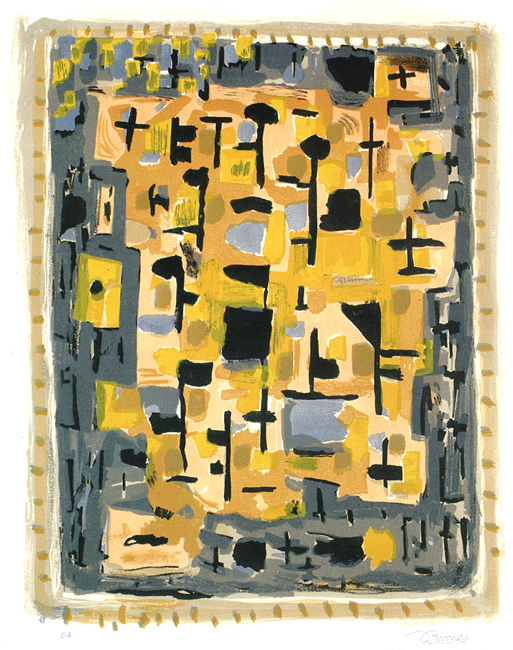This intricate and abstract piece of artwork is a vertically aligned rectangular painting, framed by an alternating brown and white, notched paintbrush-style border. Just inside this, there's a gray border that lines the top and sides. Dominating the center of the painting, the background is a bluish-gray shade filled with a dynamic array of colors and shapes. The primary hues are yellow, orange, light brown, medium brown, dark blue, and light blue, along with touches of tan, silver, white, and black.

The composition features numerous black lines arranged in various forms, including crosses, capital T's, and simple stems with dots on the ends, creating a sense of randomness and structure simultaneously. The upper left corner is notably marked by several yellow blotches set against the dark blue background, resembling abstract reflections or elements of water. While there are shapes that might remind one of lampposts, flags, or markers, the interpretation of these forms is left up to the viewer, as it is an abstract design without any discernible objects or text. The painting, replete with its vibrant and contrasting elements, covers the entirety of the image, embodying a style worthy of display in an art show.